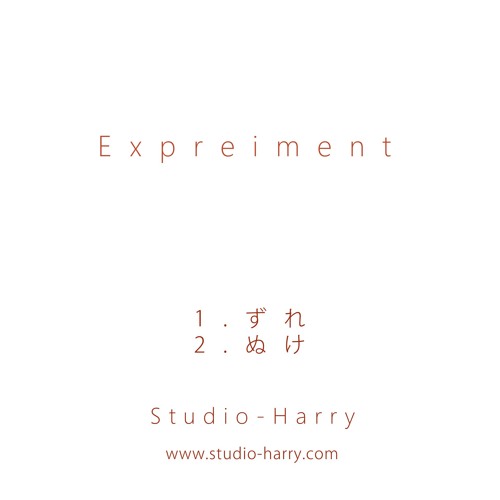The image is a simple poster with a completely white background and thin brown text. At the top, it prominently features the word "EXPERIMENT," misspelled as "E-X-P-R-E-I-M-E-N-T," with each letter spaced apart. Below this, around the center of the poster, there are two lines of text: the first line begins with the numeral "1." followed by two Japanese characters, and the second line starts with "2." followed by another set of Japanese characters. Towards the bottom, it reads "STUDIO-HARRY," and at the very bottom, there is a link: "www.studio-harry.com."